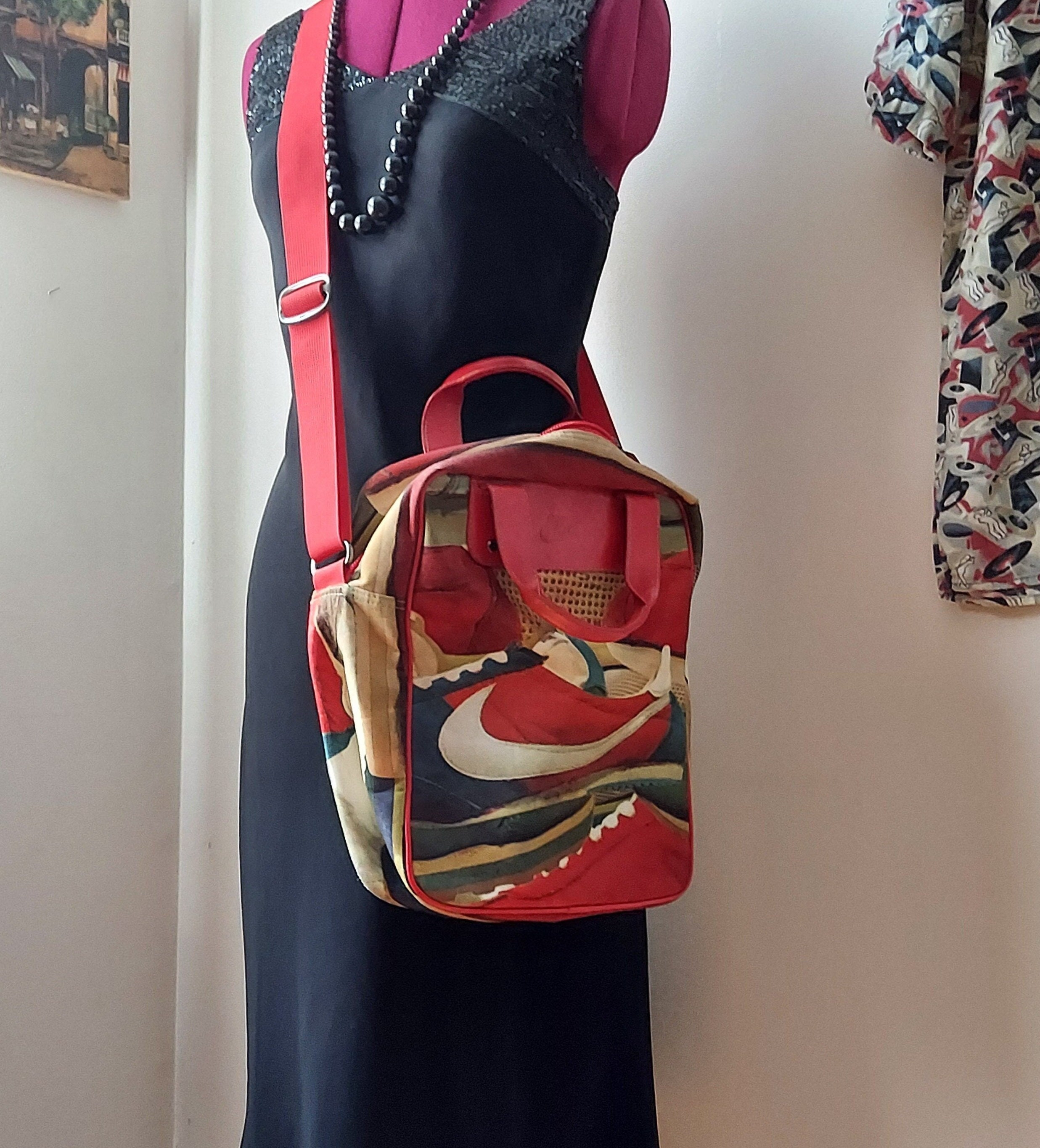This indoor photograph features a prominently positioned, armless mannequin with a violet or pink hue, tucked into the corner of the room. The mannequin is adorned in a long, sleeveless black dress that flows elegantly down its form. It showcases an eye-catching necklace comprised of large black pearls, which gradually decrease in size as they ascend towards the neck. Draped over the mannequin’s right shoulder is a distinctive cross-body bag with vivid red, blue, and green hues, which possesses a quilted design, possibly resembling a vintage camera bag or a Nike bag with an abstract pattern on the front and an orange strap. This contrasting accessory stands out vividly against the dark attire. The room features a grayish-purple wall, on which there is a framed painting alongside a hanging shirt decorated with whimsical, abstract motifs including floral elements, airplanes, and horns in shades of pink and white.